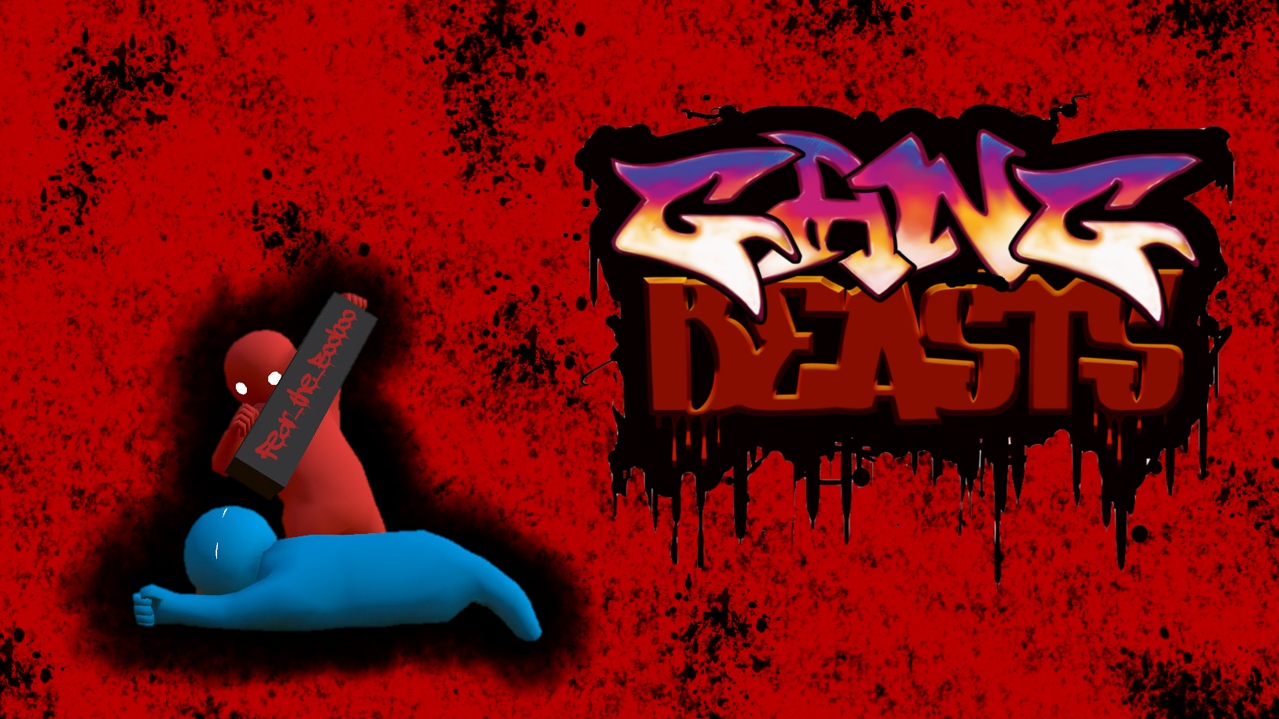The image appears to depict a screen that seems to be from an online game, though the exact nature is unclear. The background prominently features a red hue interspersed with an array of small black dots, which appear denser in certain areas, creating a textured effect. 

Towards the middle-right area of the image are the words "GANG" and "BEASTS." "GANG" is written in bold, capitalized letters with an intricate gradient effect: the top portion is a vivid blue, transitioning into a striking pink, and then a bright yellow towards the bottom, giving the appearance of illumination. Beneath "GANG" is the word "BEASTS," also in capitalized letters, entirely in red. The lettering has a background of solid black, which seems to be dripping at the bottom and along the sides, enhancing the dramatic flair.

To the left of the text, there are animated characters resembling small doughboys. One character is red with two bright, white, glowing eyes, holding a rectangular black banner. On this banner, the phrase "FEAR THE BUDDHA" is written in red. Another doughboy figure, colored blue with narrow white eye slits, lies on the ground. This figure's right arm is raised while its right leg appears to droop; notably, these figures lack detailed feet.

The overall backdrop behind these elements is black, accentuating the vivid colors and dramatic elements of the foreground imagery.